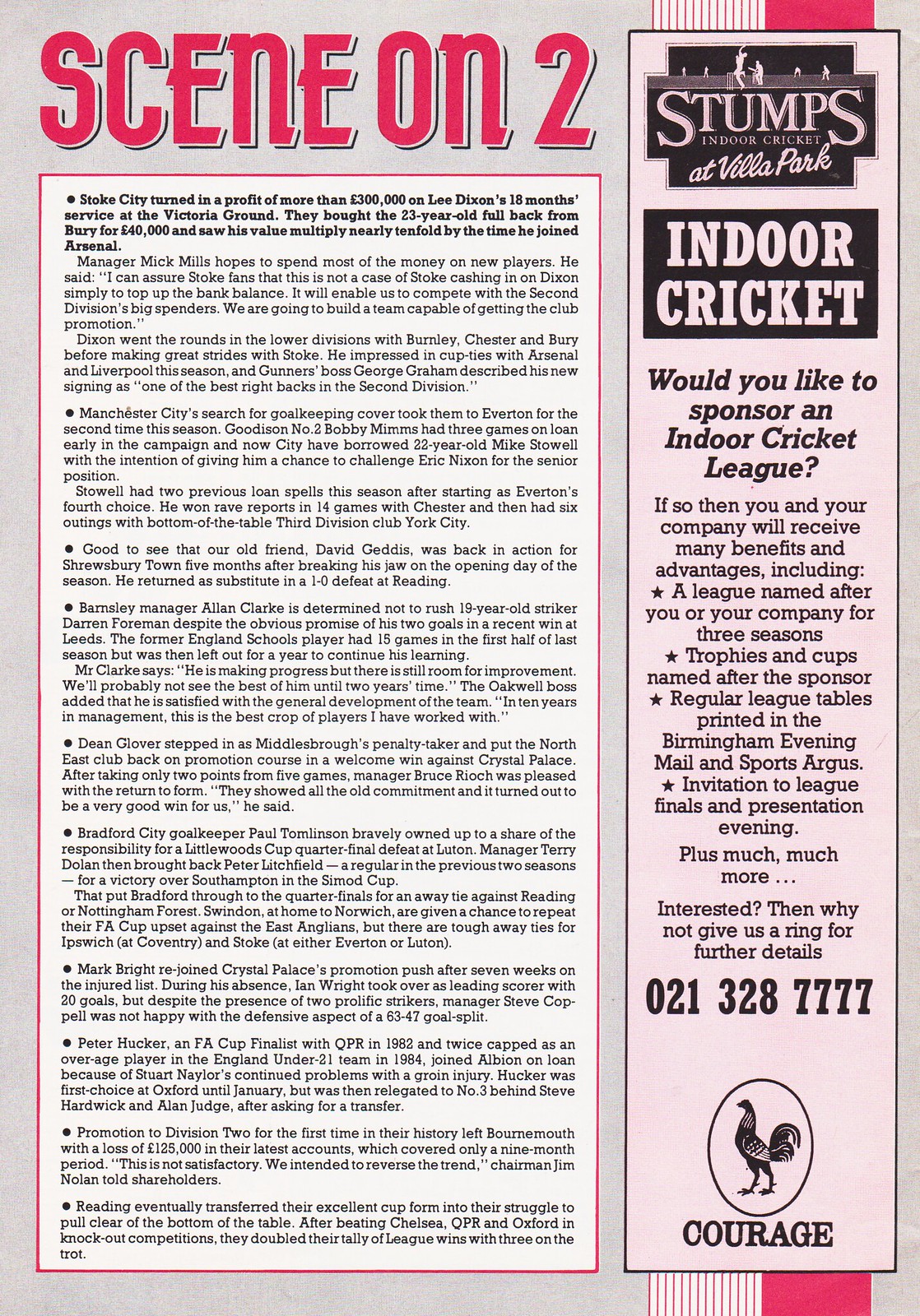The image is a page from a magazine with a predominantly gray background, featuring two distinct columns. The left two-thirds of the page is an informational section with the header "SEEN ON TWO" in bold, pink text with white shadowing. Below this, there's a white rectangular box outlined in bright pink, containing small black text in multiple paragraphs and bullet points. The top of the text is bolded and mentions that "Stoke City turned in a profit of more than 300,000 pounds on Lee Dixon's 18-month service at the Victoria Ground," indicating it is soccer-related. Details about buying the player for 40,000 pounds and selling him nearly tenfold higher to Arsenal are present, though the specifics in the smaller text are unclear due to size.

The rightmost third of the page is an advertisement for "Stumps Indoor Cricket at Villa Park." A banner with pink and white stripes on the left and bright pink on the right peeks out at the top and bottom margins. Overlaid on this banner is a black-border rectangle with a light pink background. At the top of this rectangle, a cross-shaped logo for Stumps Indoor Cricket is featured in white text on a black background. Below the logo, a smaller rectangle with "INDOOR CRICKET" in white capital letters on a black background is present, followed by promotional text in black font inviting companies to sponsor an indoor cricket league. Benefits include having the league and trophies named after the sponsor, tables printed in local newspapers, and invitations to league finals. Contact details are provided with the phone number 021-328-7777. At the bottom of this column, there is an oval image of a chicken with the word "COURAGE" in all caps beneath it, matching the column’s background color.